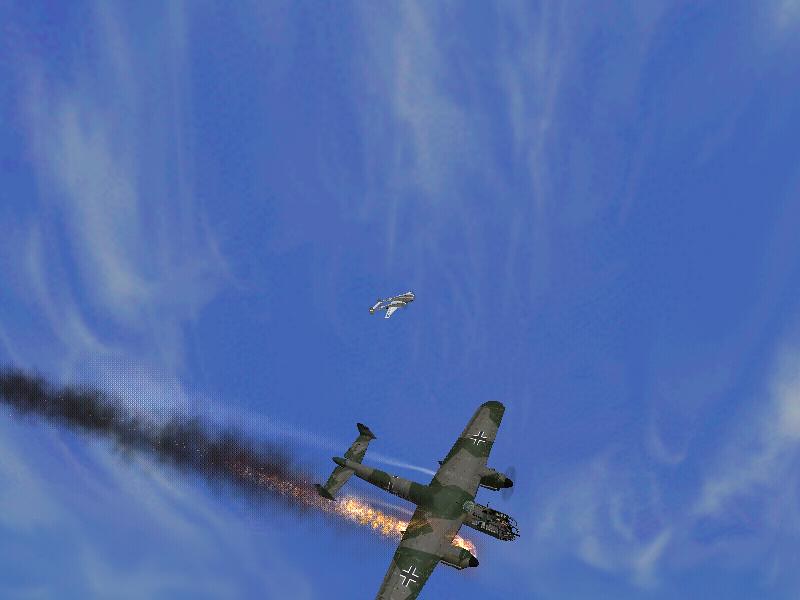The photograph captures a dramatic aerial scene set against a deep blue sky adorned with wispy cirrus clouds. The focal point of the image is a grayish-green, old-fashioned fighter plane situated at the bottom center, with its front end pointed downward in a plunging descent. Distinctive black crosses adorn each wing, marked in stylized white outlines. The right side of the plane, engulfed in bright orange flames, trails a thick plume of black smoke that stretches across the image to the left. Notably, a second, smaller gray plane hovers in the background above the chaos, barely visible against the expansive sky, adding a sense of conflict and urgency to the scene.